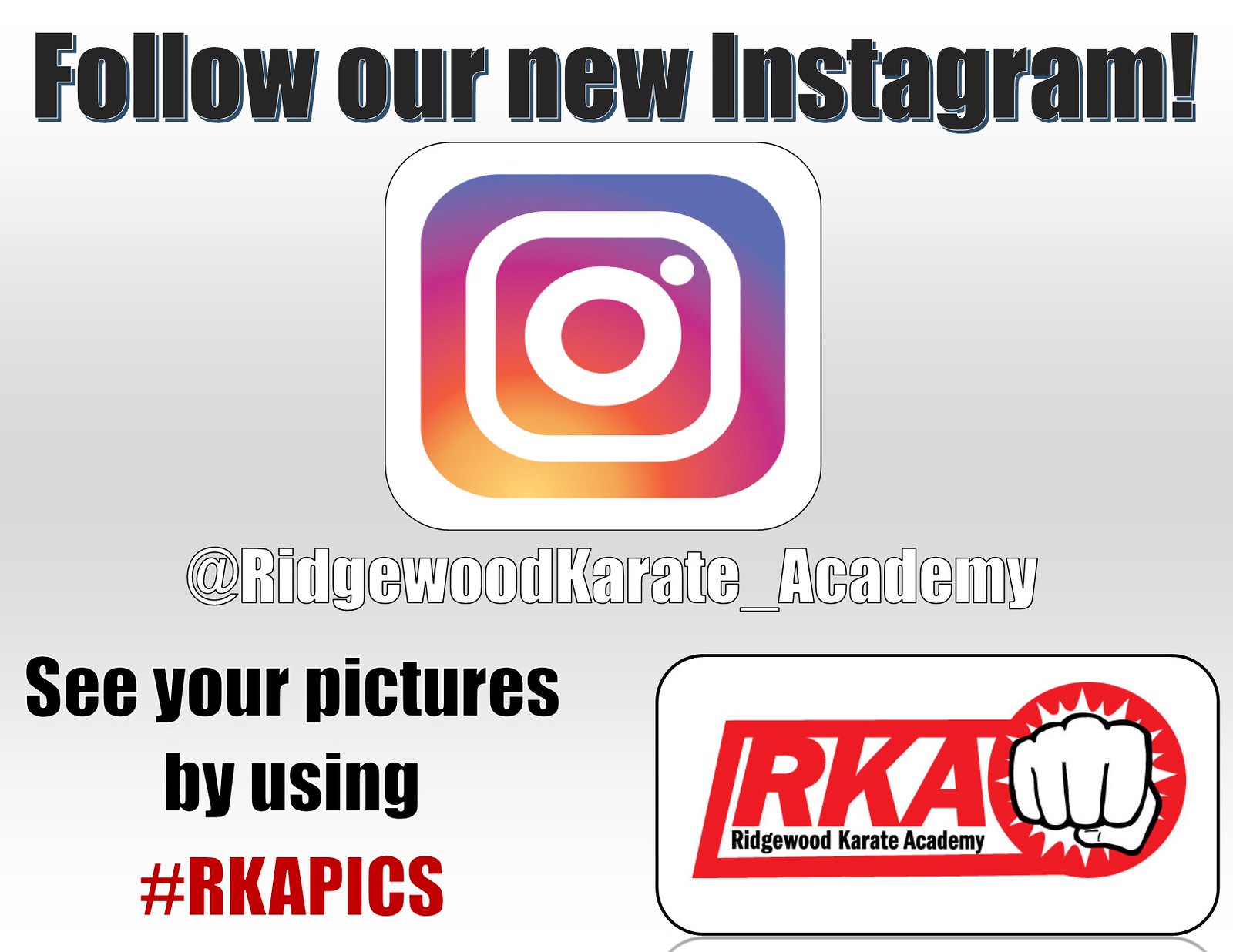The sign features a detailed and dynamic advertisement for Ridgewood Karate Academy's new Instagram account. At the very top, in large black font, the message "Follow Our New Instagram!" commands attention. Directly beneath this, prominently centered, is the iconic Instagram logo. The logo is a white square with rounded corners, containing a gradient circle that transitions from purple and pink to red, encapsulating a smaller white circle and dot in the center.

Below the logo, in white font, it reads "@RidgewoodKarateAcademy," inviting viewers to follow the account. The background of the entire sign is a muted gray, providing a subtle backdrop that makes the text and logos stand out. On the bottom left of the poster, black text encourages engagement: "See your pictures by using," followed by the hashtag "#RKAPICS" in vivid red or magenta.

To the right of this, enclosed in a white rectangular border, is the Ridgewood Karate Academy's logo. It features the letters "RKA" and a dynamic illustration of a fist, akin to a comic book punch effect, suggesting action and energy. This punch icon, partially extending from the border, reinforces the martial arts theme of the academy. This well-coordinated design effectively promotes the academy's social media presence through clear calls to action and vibrant visuals.